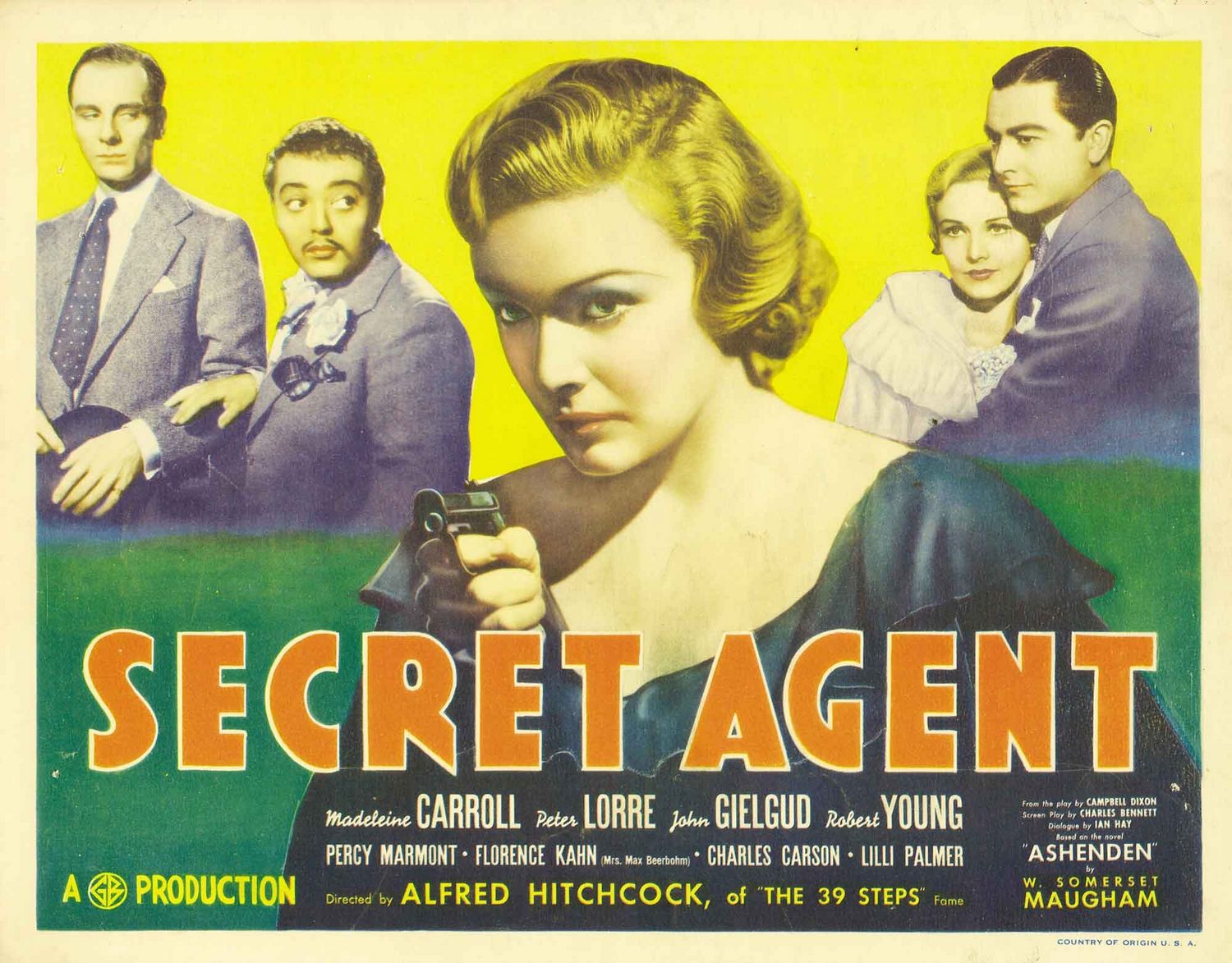The vintage movie poster from early Hollywood advertises Alfred Hitchcock's film "Secret Agent." Dominating the center is a fair-skinned, blonde woman with wavy, chin-length hair, gripping a small gun in her right hand. She is dressed in a navy blue v-necked top adorned with two ruffles. The background blends from a yellow band at the top to a green band at the bottom, creating a visually striking contrast. 

To her left are two men, both in suits; one holds his hat in his hands, while the other sports a flower on his lapel, both looking sideways with an air of concern. On her right, in the yellow band, is a couple—a man with short brown hair, dressed in a suit, embraces a short-haired young woman in a white ruffled top.

Bold orange lettering splashed across the woman reads "SECRET AGENT," with white font below listing the actors and actresses. Further details about the production and direction by Alfred Hitchcock appear in yellow lettering at the poster's bottom.